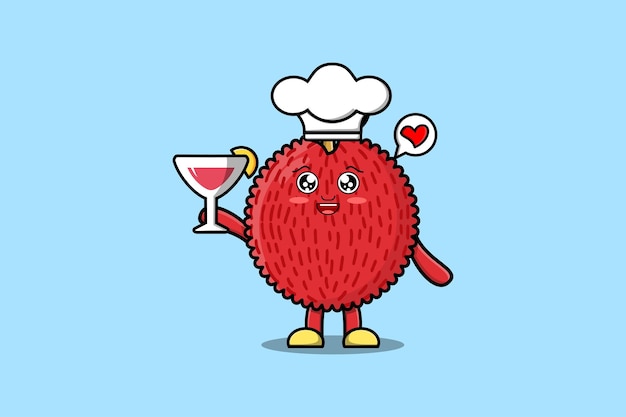In this cartoon image set against a light blue background, we see a charming and vibrant character that resembles a fuzzy red raspberry or fluffy berry, with distinct raspberry-like textures and red lines suggesting a fuzzy appearance. This animated fruit stands out with its big, round, anime-style eyes adorned with reflective white dots, lending a perpetually happy and joyful expression. The character sports a cheerful smile and rosy cheeks, enhancing its endearing presence. 

Atop its head is a white chef's hat, adding a whimsical touch to its overall look. Completing the ensemble, the character wears bright yellow shoes. In its hand, it holds a clear glass filled with a red or pink cocktail, possibly a cosmopolitan, garnished with a lemon wedge on the rim. The detail and vibrant colors of the drink add to the lively nature of the image.

To the right of the character floats a thought bubble with a big red heart, suggesting feelings of love or happiness. This delightful berry-like figure is clearly in high spirits, radiating positivity and charm in its animated, computer-generated form.